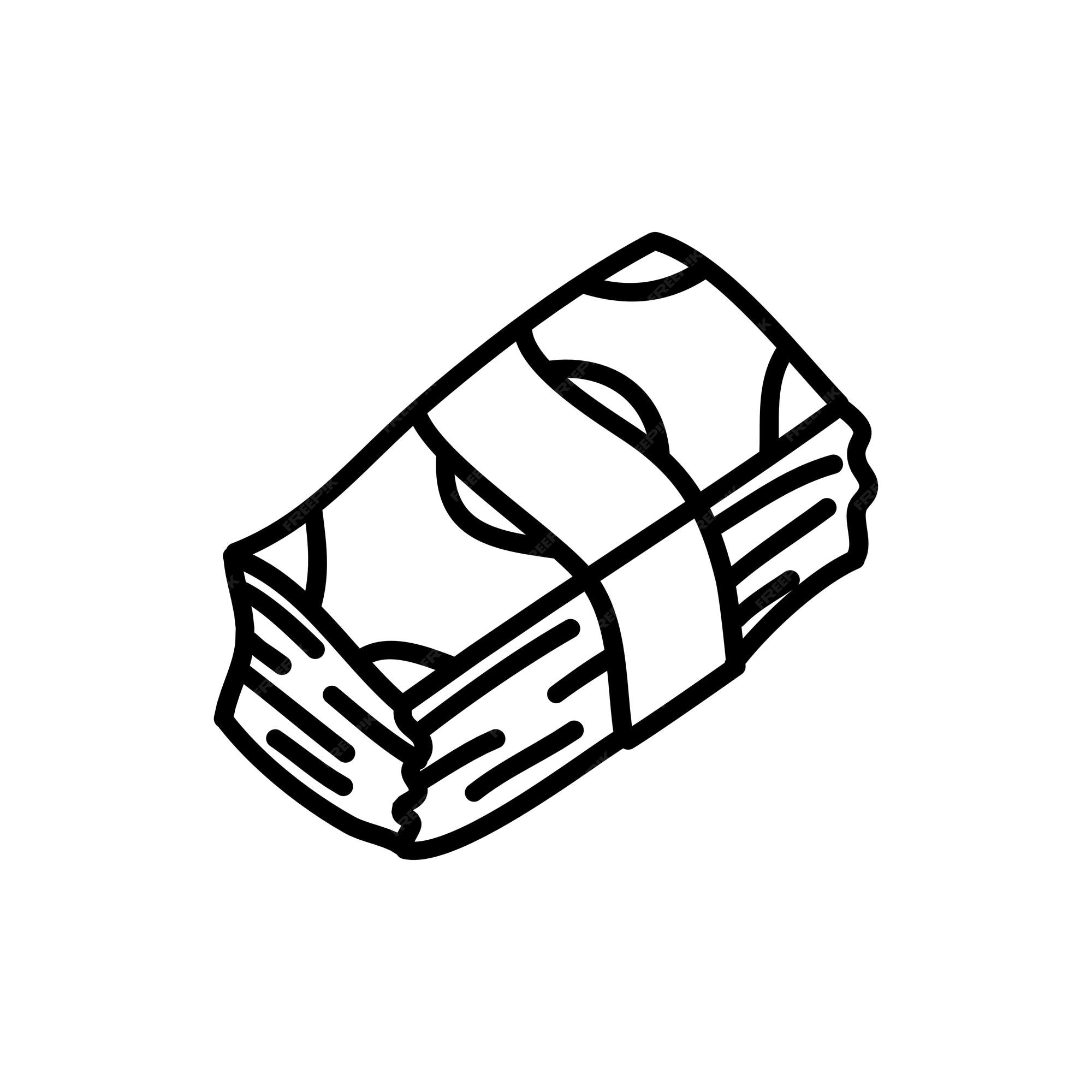This image depicts a simple, black-and-white cartoon-style illustration of a stack of money. The stack, shown in a slightly diagonal orientation from the bottom left to the top right, is detailed through uniform thick black lines. The stack is bound together by a white paper money holder, commonly seen in banks for organizing currency. The depiction includes horizontal lines to indicate multiple bills within the stack, and a single bill's face, partially obscured by the paper holder, has quarter semicircles at each corner and a circle in the center. The entire illustration is set against a plain white background, with no specific currency or denomination identified.